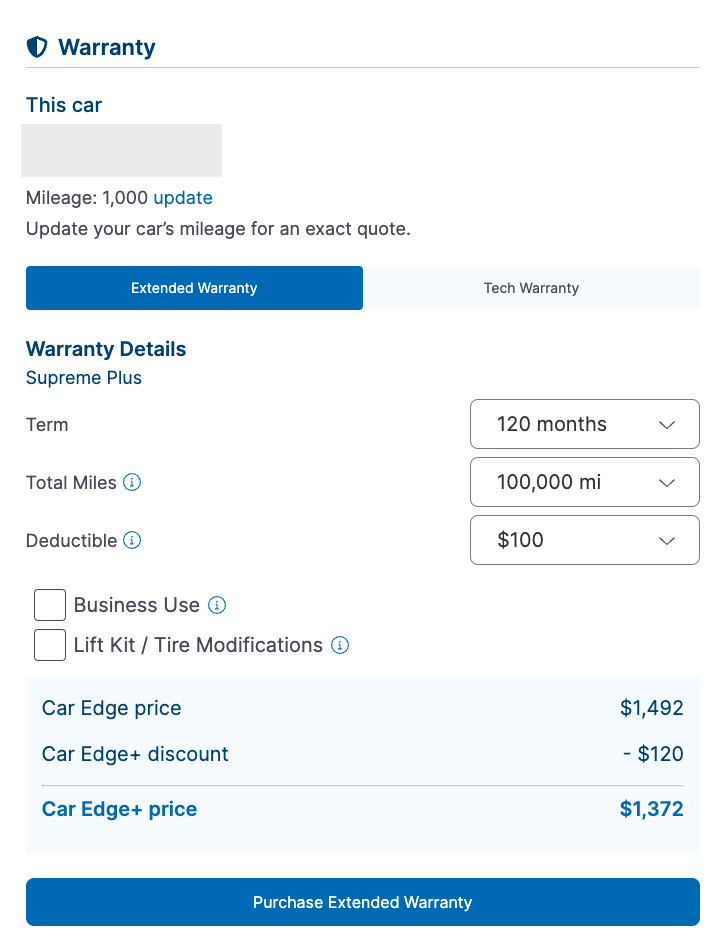Detailed caption:
---
The image is a screenshot featuring a car warranty document. In the upper left-hand corner, the word "Warranty" is prominently displayed next to a shield symbol. "This Car" is written below, followed by a redacted gray box. Beneath this, "Mileage: 1000" is shown with an option to update the mileage, accompanied by the prompt, "Update your car's mileage for an exact quote."

The document features two warranty options: "Extended Warranty" and "Tech Warranty," with the "Extended Warranty" option selected. Underneath, it specifies, "Warranty Details" with the type listed as "Supreme Plus."

Details under this section include:
- Term: 120 months 
- Total Miles: 100,000 miles
- Deductible: $100

Pricing information provided includes:
- Car Edge Price: $1,492
- Car Edge Discount: -$120
- Car Edge Plus Price: $1,372
---